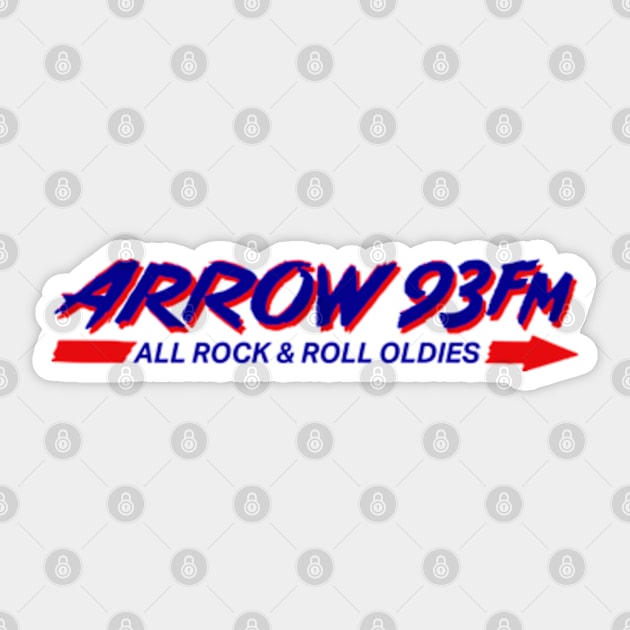This image is a digital advertisement for a radio station, prominently featuring a bold, three-dimensional design. It is large and square with a light gray background, adorned with thin gray lines forming a grid of square shapes. At the intersections of these lines, there are darker gray circles, each containing an image of a white padlock. 

At the center of the image, stretching horizontally from left to right, is the main focus: large, bold italic text in dark blue with a jagged three-dimensional effect, accompanied by a red drop shadow, spelling out "Arrow 93 FM." Below this, in the same dark blue font, are the words "all rock and roll oldies," positioned within the center cutout of a red arrow that points to the right. This central section of text and arrow is set against a white background strip that runs horizontally across the image.

Overall, the advertisement is vibrant with its prominent use of royal blue and red against the grayscale backdrop, which features a repeated pattern of padlocks in a circle. The style reflects a photographic realism of a printed decal or sticker applied onto a digitally created background, effectively drawing attention to the radio station's branding.